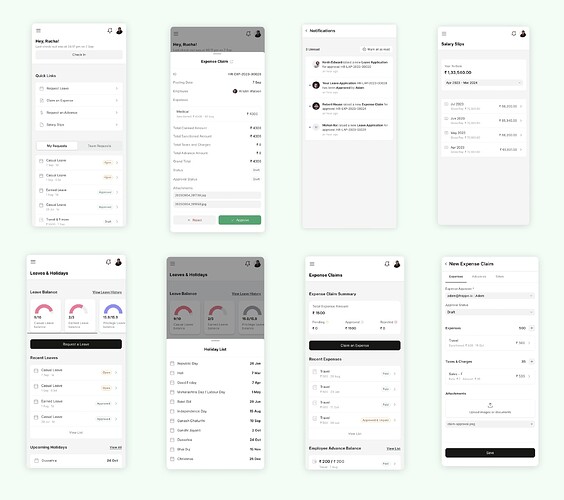The image features eight small screen captures from a smartphone, each arranged in a compact grid. Due to their diminutive size, the exact content of these screens is difficult to discern. However, two of these captures stand out, each displaying pie charts rendered in vibrant colors. These pie charts contain three distinct sections apiece. The remaining six screens exhibit a variety of text readouts in monochromatic shades of gray, white, and black, all of which remain illegible. Each screen is distinctly shaped to mirror the typical contours of a smartphone display. There are minimal additional details at the top portions of the phones, maintaining a focus on the contents of the screen.